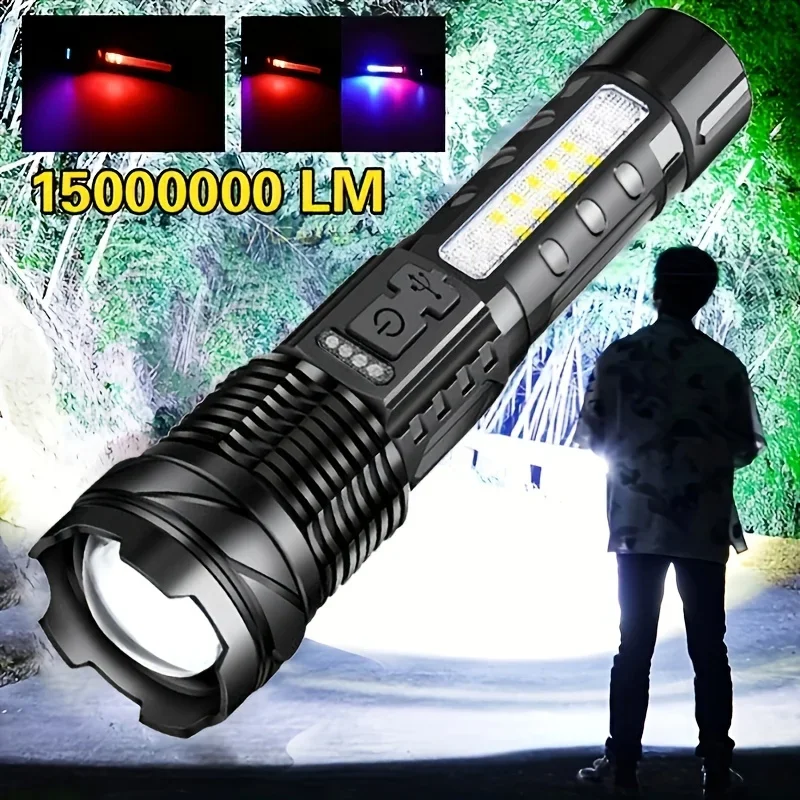The image is an advertisement for a black flashlight, designed with a power button and a light strip on the handle, which is made of a mix of metal and plastic. The flashlight, fairly skinny and diagonally positioned with its light bulb pointing downwards, is shown emitting an intense beam in a forest-like background filled with green trees. The brightness of the flashlight is emphasized by the overexposed white light it casts, illuminating the area and a person standing on the right side, slightly obscured by shadows. In the upper left corner of the image, two smaller photos display the flashlight's light strip feature, accompanied by a yellow text with a black outline that reads "1500000LM," indicating the flashlight's impressive lumen rating of 15 million lumens.